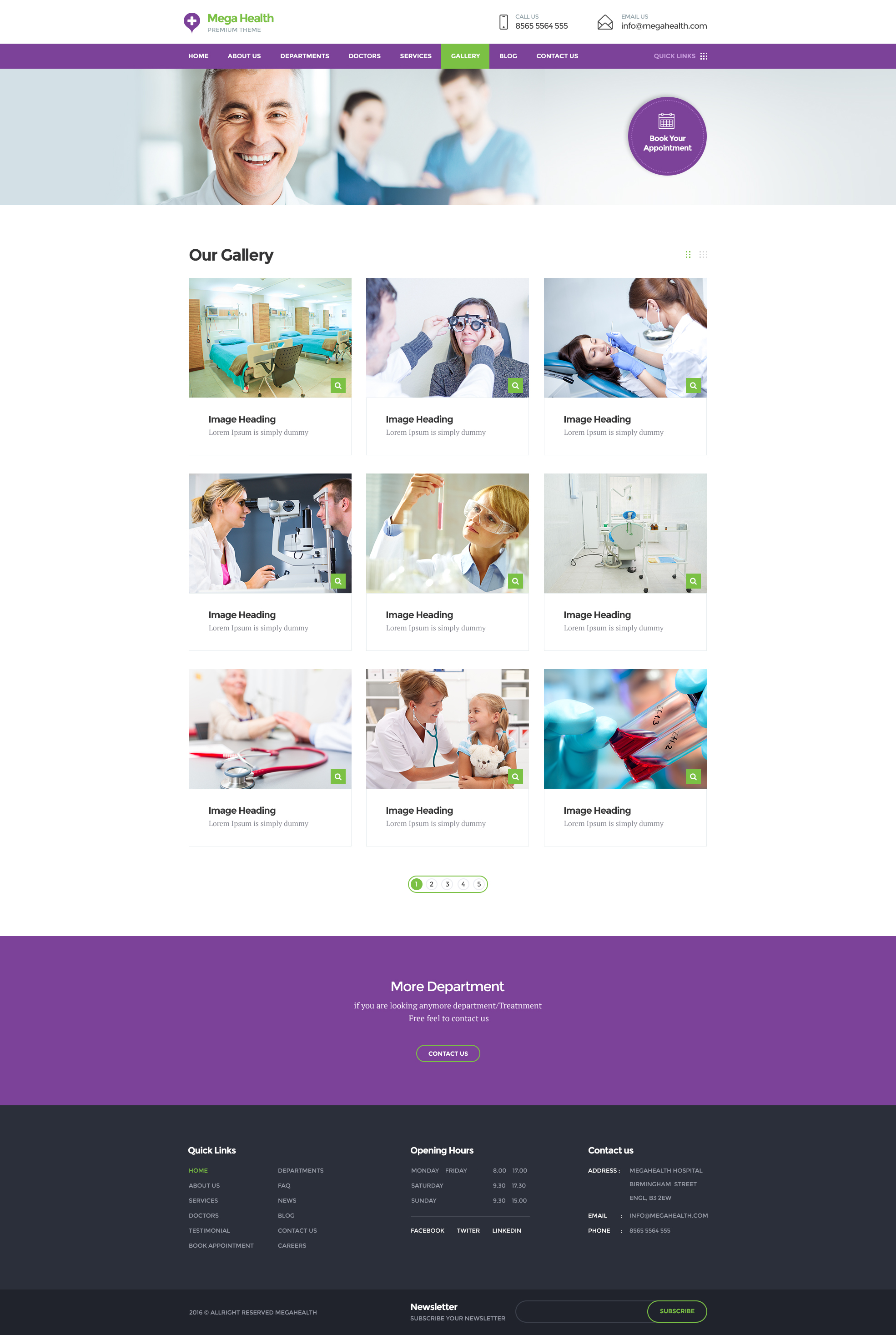The image depicts a healthcare website viewed from a distance, making the text difficult to read. At the top, the site title, possibly "Mega Health," is displayed in green lettering. Below the header, there are some illegible options. A contact section is visible, accompanied by a picture of medical professionals. There is a clickable circle, with the label "Our Gallery" underneath it, leading to a triplet of image boxes, each linked to different content. Further down, there are three more images of medical professionals, followed by another set of three clickable boxes showcasing various medical areas. At the bottom, the page lists multiple departments with additional contact information, and the standard sections found on most websites such as "Contact Us" and other navigational links.